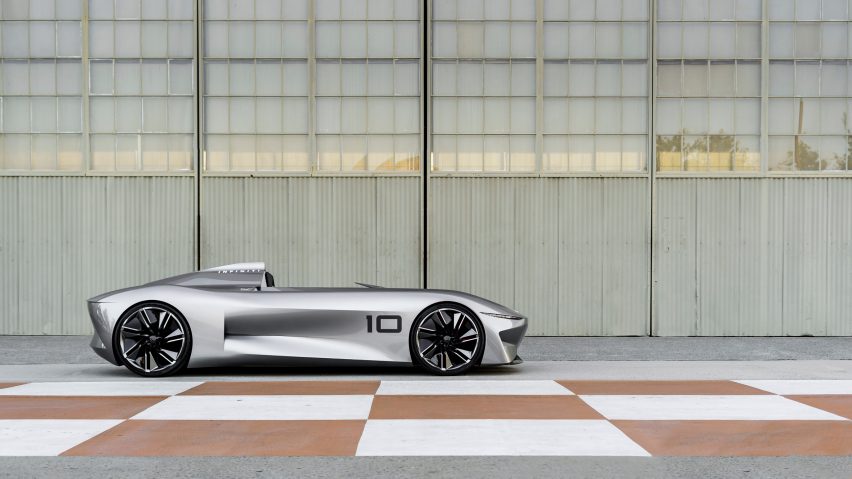In this captivating photograph, a sleek and futuristic silver convertible roadster, marked with the number 10, is prominently featured in front of a building that resembles a warehouse or hangar. The building has light green panels and large, hanger-like doors, with a series of small, square windows above. These windows reflect a yellow building across the street. The surface on which the car rests is a distinguishing red and white checkered pattern, creating the illusion of a racing start or finish line. The car, low to the ground with a streamlined design, exudes a modern, almost concept-car vibe, evoking images of a vehicle from a futuristic movie. Performance tires and the highly polished, metallic exterior add to its sophisticated appearance.